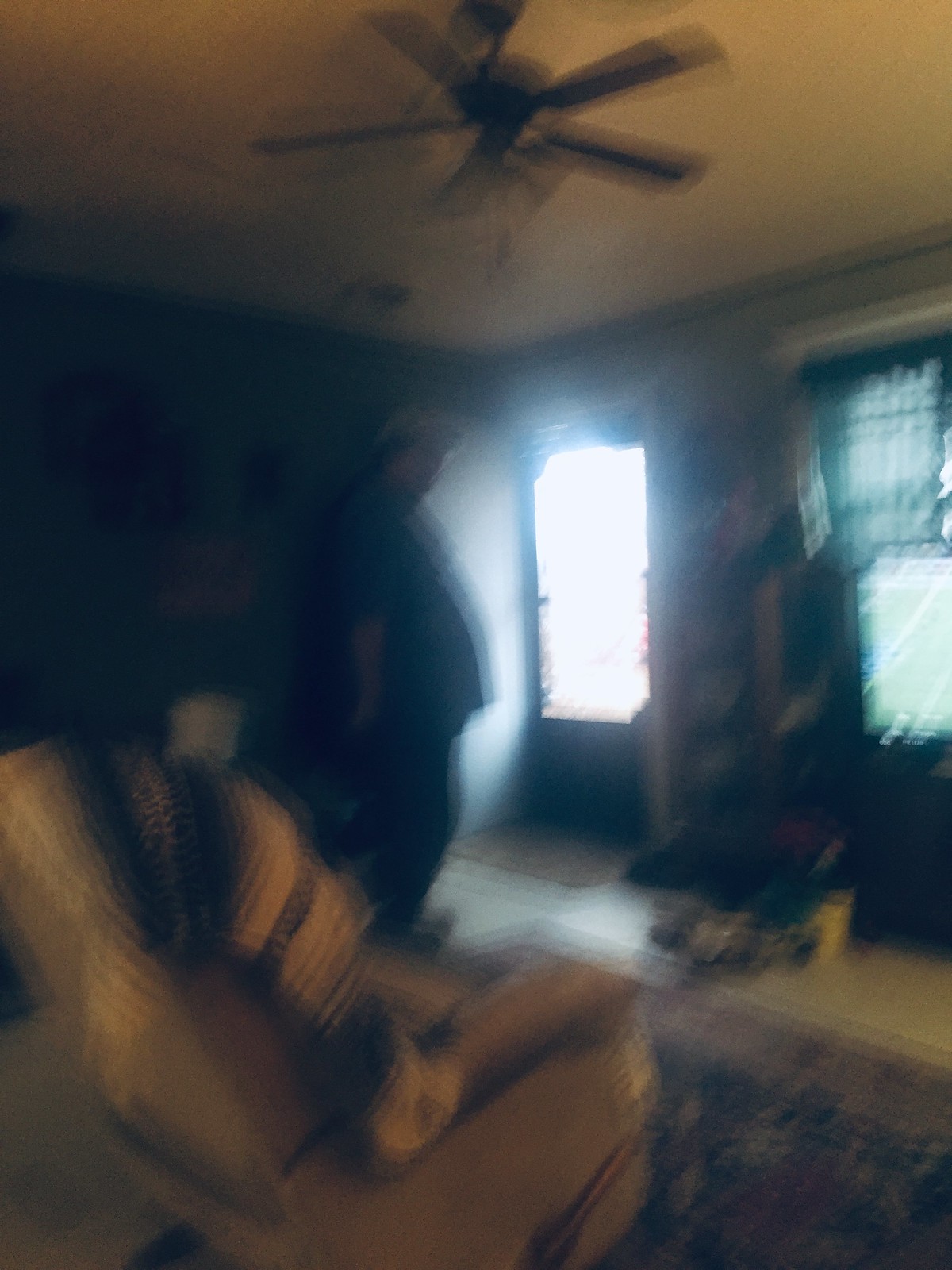In this somewhat blurry image of a living room, the central focus is on a man with black hair, wearing a white hat. He appears to be somewhat large in stature and is dressed in a long, dark green shirt paired with dark pants. The man is facing to the right. Mounted in the center of the ceiling, directly above him, is a ceiling fan. In the foreground, there's a light brown or light gray recliner draped with a blanket. Beyond the man, the front door is visible, partially open, with a mat on the floor beside it. The door features a glass panel, allowing an abundance of natural light to flood into the room.